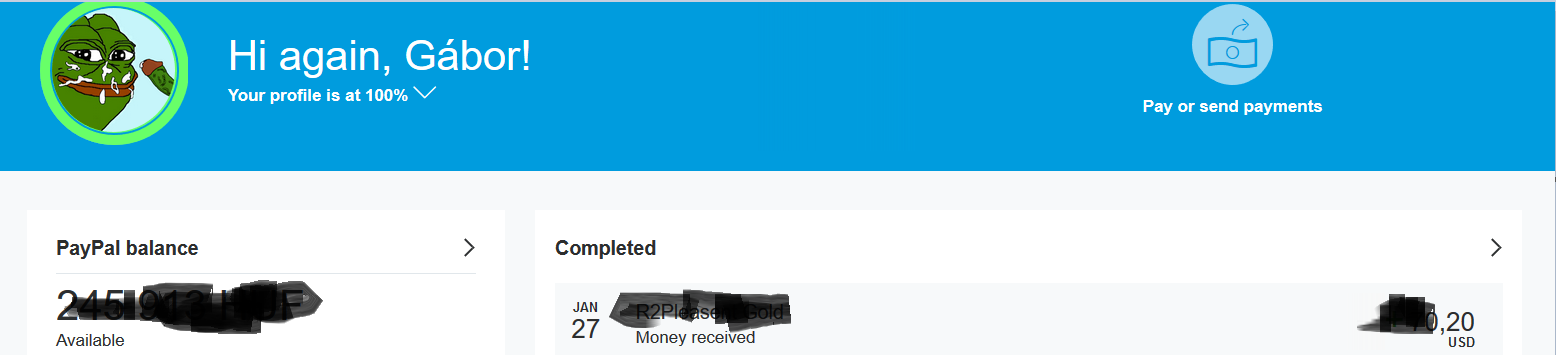A screenshot of a PayPal account interface is shown, featuring a user named Gabor, reminiscent of the iconic Gabor sisters. The prominent profile picture is a whimsical cartoon monster featuring shades of blue and white. Most of the financial details, including the account balance and transactions, are obscured as if marked out for privacy. Visible within the image is a single transaction indicating $20 USD received on January 27th. The interface displays typical PayPal colors – a mix of blue, green, black, and white. The overall display appears to be a close-up, possibly taken from a smartphone or tablet, revealing the user's account status, which is 100% complete for sending and receiving payments.